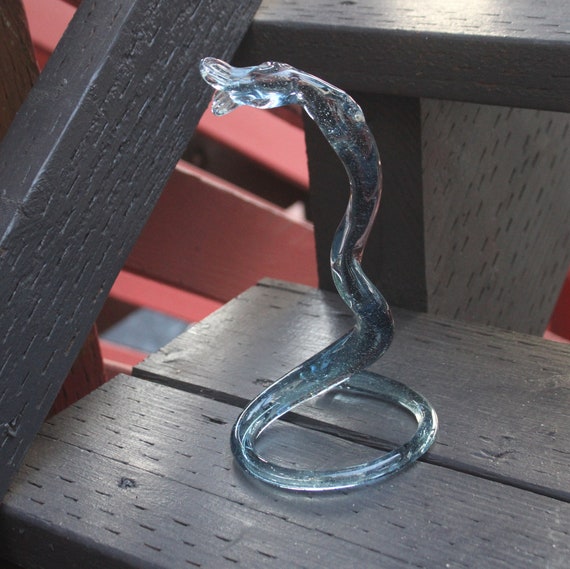This photograph captures a translucent, clear, plastic-like sculpture resembling a snake, situated on a dark gray outdoor step. The sculpture, seemingly crafted from plastic, acrylic, or resin, exhibits a pale blue color. Notably, the sculpture's coiled base forms a circle, enabling it to stand upright. Bubbles are suspended within the see-through material, adding to its intricate design. The snake-like figure spirals upwards, evoking the image of a snake poised to strike. Despite its delicate, tall, and thin structure, details such as the small crystals within the material and the possible subtle facial features, like an eye and a mouth that resembles a fish's, amplify its lifelike appearance. The scene is illuminated by daylight, with the sunlight casting a subtle glow on the step above. In the backdrop, a burgundy-colored wooden surface, perhaps another set of steps, adds a contrasting depth to this close-up outdoor photograph.